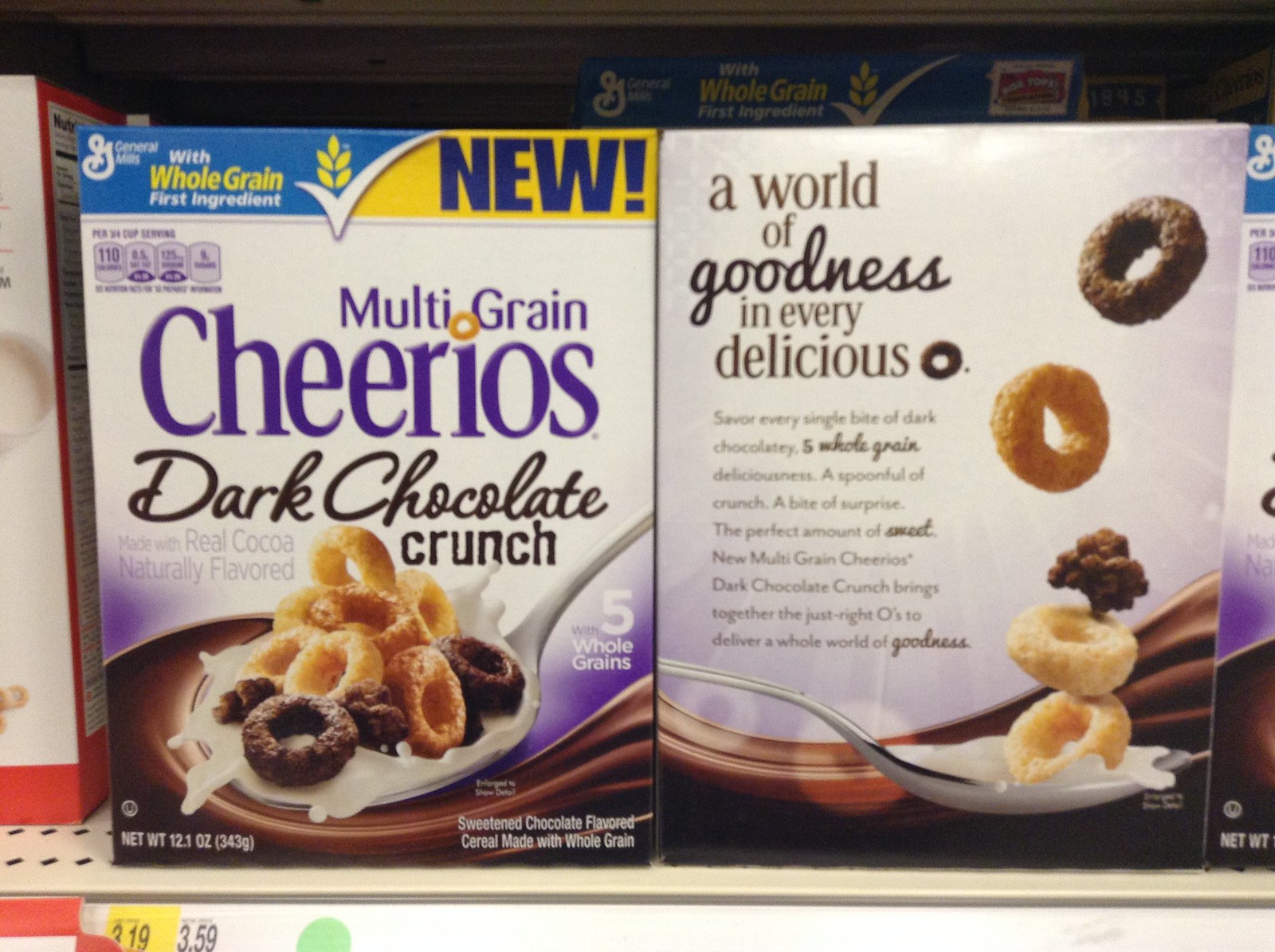This image is a detailed photograph taken in a grocery store aisle, focusing on boxes of Multigrain Cheerios Dark Chocolate Crunch cereal placed on an off-white beige metal shelf. The shelf features numerous small holes and has price tags displayed at the bottom left corner: $3.19 highlighted in yellow and $3.59 next to a green circle. Dominating the image, the left cereal box is facing forward, showcasing the General Mills branding in the top left and a spoon filled with cereal pieces in various shades of brown splashing in milk. The packaging emphasizes that whole grain is the first ingredient and labels it as a new product. Adjacent to this, the right box reveals the back design, headlined with, "A World of Goodness in Every Delicious O," displayed alongside large Cheerios falling into a spoon of milk. Behind the two primary boxes, the tops of additional Multigrain Cheerios boxes are partially visible. Off to the left edge, just within the frame, another distinct cereal box is barely seen.